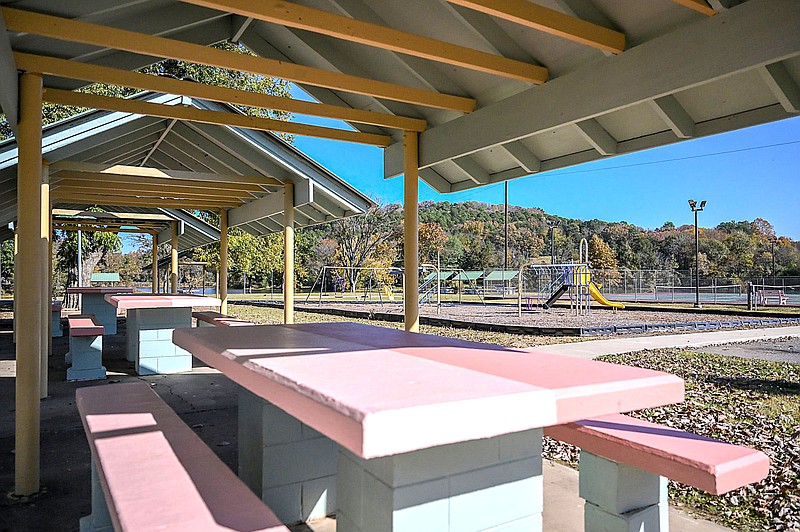This color photograph captures a vibrant outdoor scene at a public park, likely situated in the United States. The image prominently features three wooden shelters, each boasting a roof supported by light brown pillars. Positioned under these structures are concrete picnic tables, uniquely painted in varying shades of pink—light pink on one side and dark pink on the other, with matching benches. 

In the foreground, the shelters are spaced apart, providing shaded areas for visitors. Moving beyond these shelters, a well-equipped playground stretches out across the scene, set on a bed of wood chips. This playground includes a yellow slide, silver-gray monkey bars, swings, and a merry-go-round, all enclosed within a fenced area. Adjacent to the playground, there are also tennis courts and possibly a basketball court, with solar panels visible in the distance.

In the background, a hill adorned with trees adds a natural touch, indicating early fall with foliage still on the branches. The sky overhead is a clear, bright blue, suggesting the photo was taken during daytime, either in the morning or afternoon. Scattered stones and a concrete sidewalk connect the picnic area to the playground, enhancing the park's accessibility and structure. The detailed composition not only captures the park's amenities but also hints at a serene, inviting atmosphere perfect for outdoor activities and leisure.